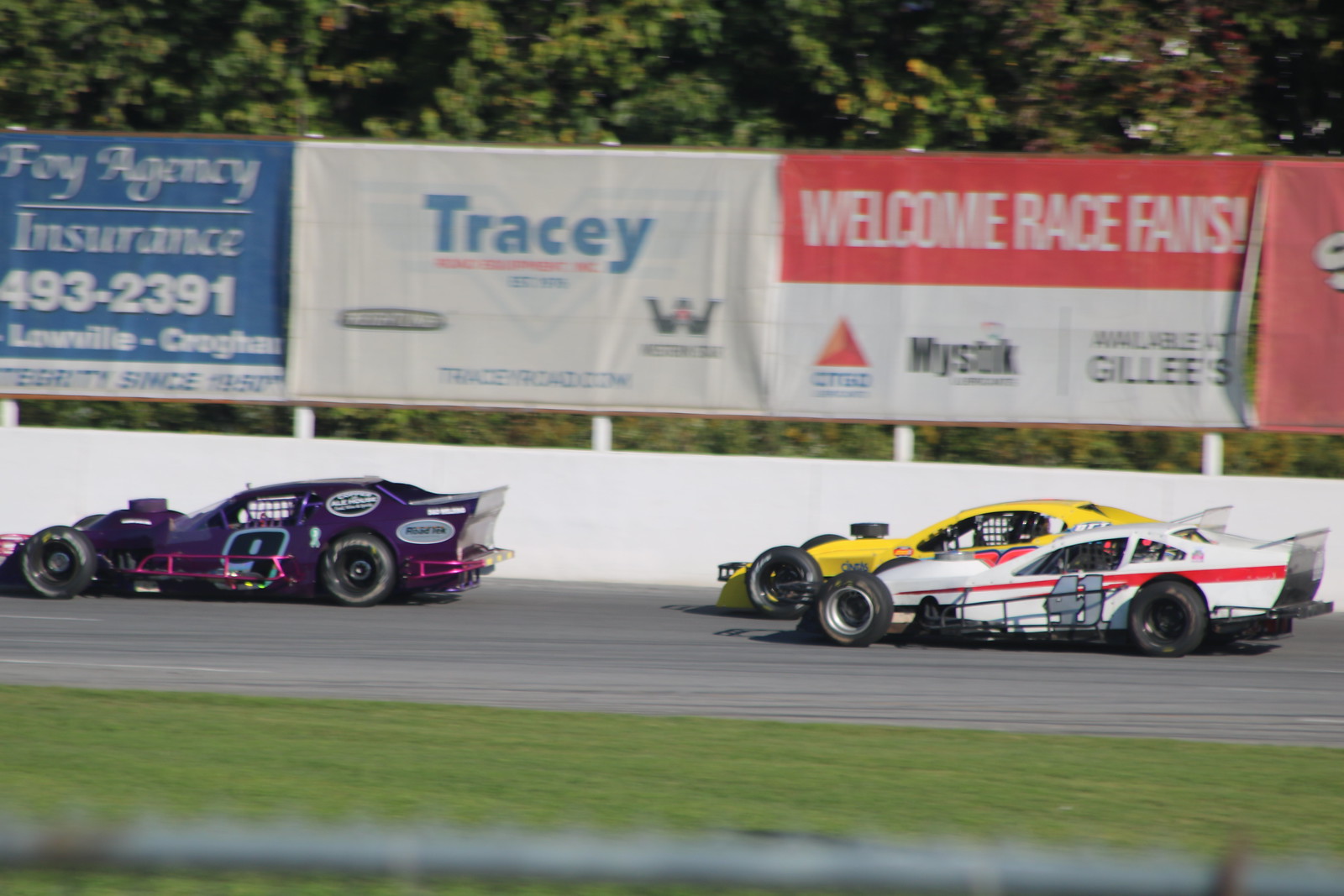This image captures a dynamic moment on a race car track, showing three unique race cars in action: a dark purple car with a prominent black number 9 leading the pack, followed by a yellow car and a white car with a red stripe and the number 41. The gray track is bordered by a white barrier, beyond which several advertisement billboards are visible. The leftmost billboard is blue with white letters reading "Foy Agency Insurance." Next to it is a billboard with a white background and blue text that says "Tracy," featuring a website URL, though it is somewhat blurry. Further right, there is a banner that greets spectators with "Welcome Race Fans." The foreground of the image includes a flat grassy area that slopes slightly downward, and a blurry gray pole-like object crosses diagonally at the very bottom. Greenery is visible behind the billboards, giving context to the race’s likely American setting.